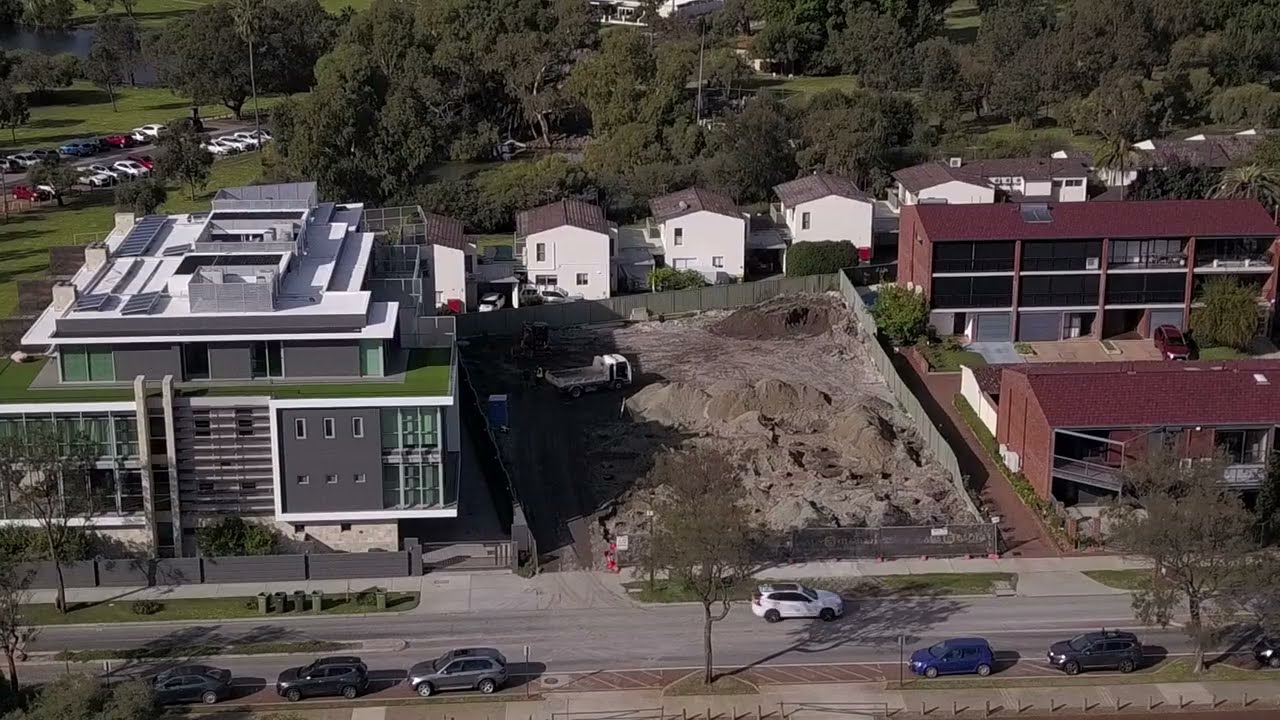The image depicts an aerial view of a neighborhood street, showcasing an active construction site between two prominent buildings. On the left, there's a large gray building with white trim, characterized by its wide and tall structure, possibly spanning multiple floors. To the right, there's a red building that appears to be residential or perhaps a commercial apartment building. The central focus is the construction site between these buildings, featuring an open dirt space where a white truck can be seen moving dirt next to a blue and white port-a-potty. The site is enclosed by a metal fence.

In front of the construction area, along a gray road lined with a light brown sidewalk, numerous cars are parked, facing left. These include dark gray, light gray, and blue vehicles. On the road itself, a white car is traveling to the right. To the left of the gray building, there's a parking lot with various cars, including white, red, and blue ones, parked in neat rows.

Behind the construction site, there's a row of white buildings with gray roofs, each potentially serving as apartments or homes. This area is framed by a large grassy space populated with tall, bushy green trees. Across the street from these buildings, one can see additional trees and another red building with a long driveway, bordered by a white fence and some trees, enhancing the residential feel of the neighborhood.